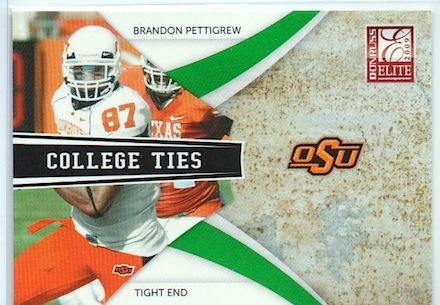This is a detailed 2009 Donruss Elite college football trading card featuring Brandon Pettigrew from Oklahoma State University (OSU). Positioned in the top right corner of the card, there's a red box with white text that reads "Elite 2009." Dominating the left side of the card, Pettigrew is captured in action wearing a white jersey with the number 87, paired with a white helmet and orange pants, suggesting a dynamic play on a football field. Behind him, a player in an orange Texas jersey and helmet is partially visible. The design includes a striking "College Ties" banner in white text on a black background running across the center of the image. Confirming Pettigrew's role, the bottom section of the card lists his position as “Tight End.” The card is further accentuated with green stripes over a white background and a textured cement-like surface, adding depth to the aesthetically-pleasing layout, all encased in a clear plastic card protector.